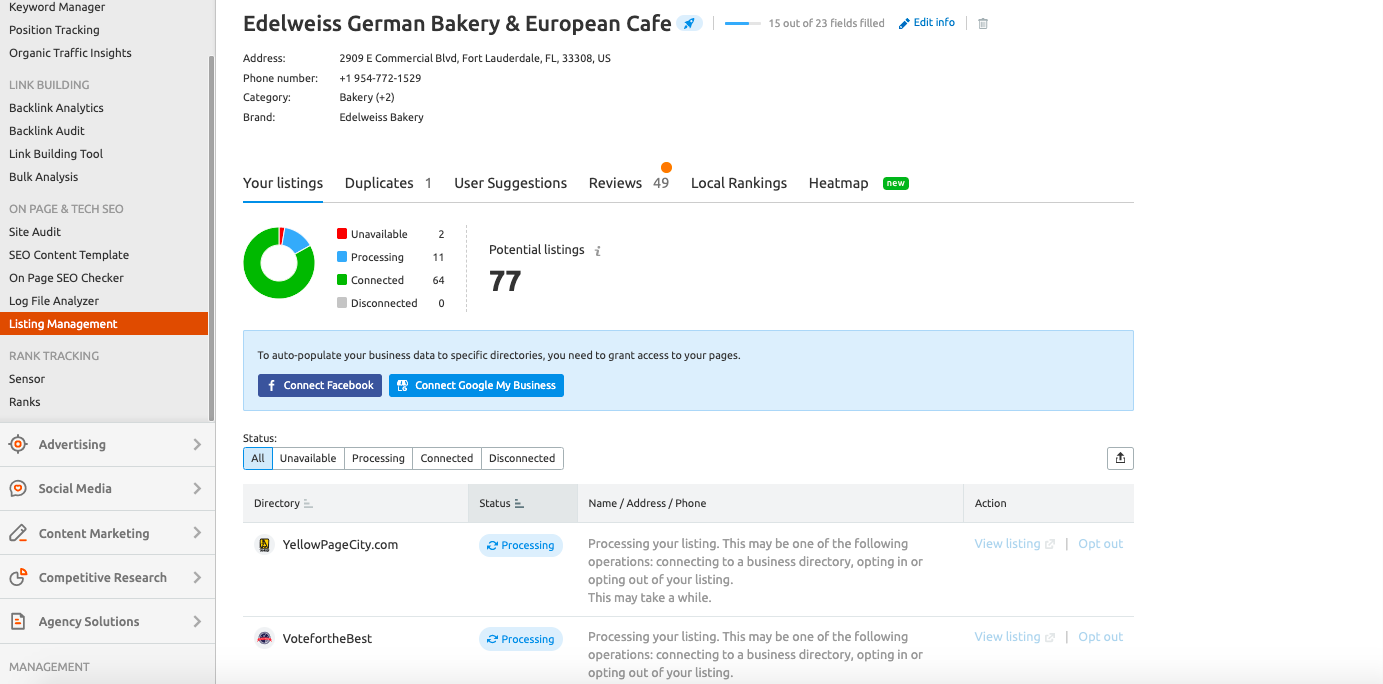This image showcases Edelweiss, a charming German bakery and European café. Renowned for its warm and inviting atmosphere, this establishment has garnered numerous user reviews and high local rankings. The bakery is easily identifiable on Google and Facebook, ensuring accurate details for potential visitors. The image's heat map indicates a significant influx of locals and tourists alike, making it a popular spot. Detailed listings and maintenance efforts are reflected in the comprehensive log file analysis.

Various behind-the-scenes tasks such as backlink analysis, site ranking, and link building are meticulously managed to boost online presence. The café's digital footprint is carefully curated through targeted advertising and social media engagements, enhancing its reach and consent among the audience. Additionally, local traffic reports suggest that Edelweiss is a favored stop for commuters and wayward passengers, contributing to its bustling environment.

On the left-hand side of the image, there's a scroll bar that likely incorporates advertising and social media updates related to the café. Overall, the picture paints a vivid and comprehensive depiction of Edelweiss, illustrating its operational nuances and vibrant customer engagement.